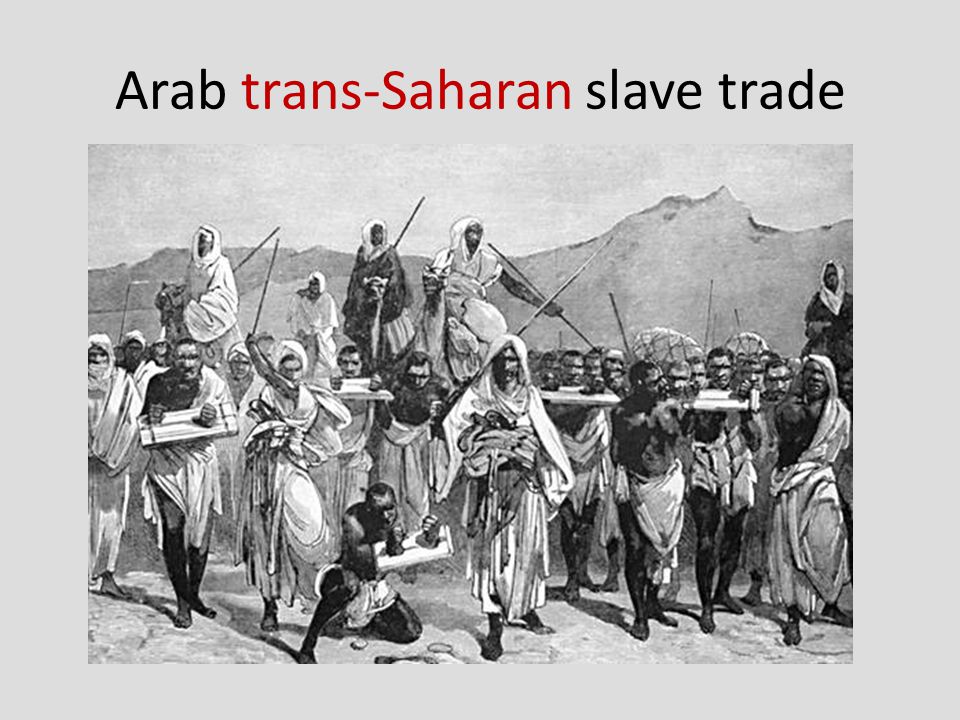The black and white illustration depicts the Arab Trans-Saharan slave trade, with the words "Arab" and "slave trade" printed in black and "Trans-Saharan" highlighted in red at the top. In the foreground, a group of black slaves, scantily clad in loincloths, are shown with their hands shackled either with boards or chains. One slave has fallen to his knees, and a white or Arab slave trader stands behind him, poised to strike with a cane or staff. Central to the image is a taller Arab figure, presumably a leader, flanked by five Arab men, some draped in white headgear and shawls, who are mounted on camels. The background features undulating hills or mountains, rendered in gray. The illustration clearly portrays the harsh and brutal conditions of the slaves under the Arab traders.